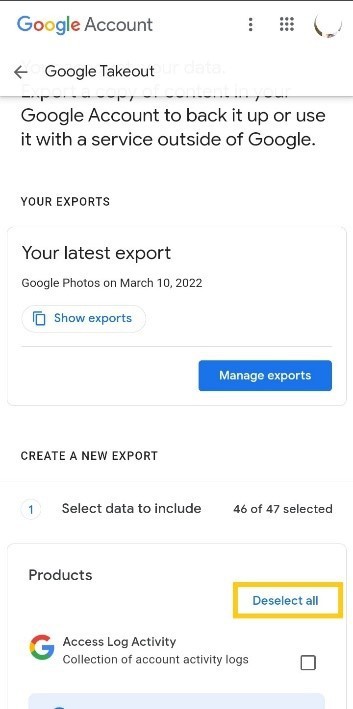This screenshot, taken from a smartphone, showcases a user's Google Account page specifically focused on Google Takeout. At the top left corner, the iconic colorful Google logo is displayed, followed by the word "Account" in gray text. The upper right corner features a row of three vertical dots next to a grid icon known as the Google Apps menu. The main section of the page has a clear white background with black text.

Prominently, large bold text reads "Google Takeout," indicating the service being accessed. Below this, an informative line explains: "Google Account to back it up or use it with a service outside of Google." Below this notice, the section titled "Your exports" is shown with "Your latest export" specifying a recent activity: "Google Photos on March 10, 2022". 

Two buttons follow: "Show Exports," in blue text, and a noticeable bright blue rectangular button labeled "Manage Exports" in white text. Moving further down, there's an option to "Create a New Export," with instructions to "Select data to include" showing that "46 of 47 selected products" have been chosen for export. 

Finally, in the lower right-hand corner of the screen, a yellow rectangular button with the text "Deselect All" is available, offering convenience for users wishing to make adjustments to their selected data.